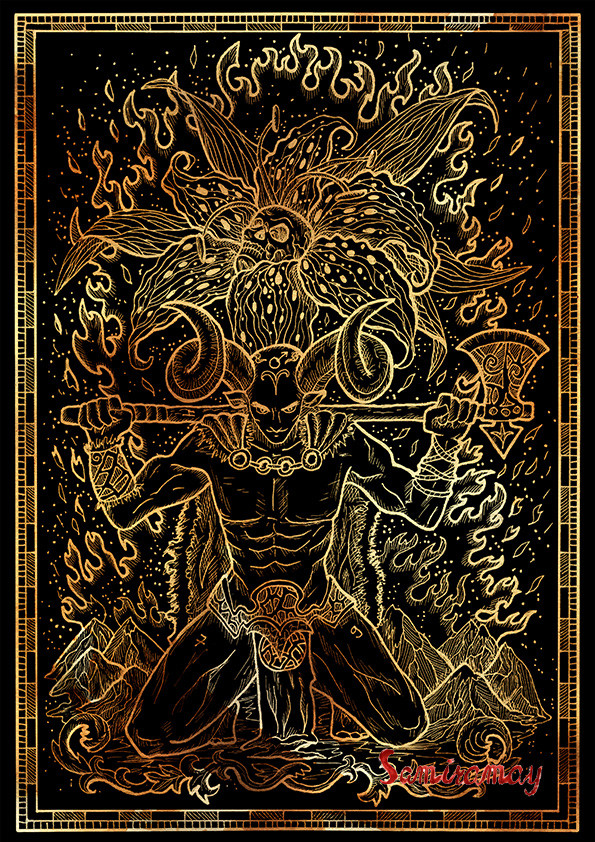This intricate artwork, predominantly in black and gold, depicts a demonic figure detailed with exceptional precision. The demon, shirtless and clad in only a cloth loincloth and a flowing cape, is kneeling with his feet tucked behind him. He boasts two long, curved horns extending from each side of his head. Balancing on his shoulders, he holds an axe with both hands behind his head. Above him, a skull surrounded by what looks like petals or leaves, resembling the center of a flower, adds to the dark, surreal atmosphere. The background features a golden border and possibly mountains, enhancing the elaborate scene. In the bottom right corner, the artist has signed the work in red, with the name 'Sam' clearly visible, although the full signature reads 'Samay' or 'Samark'. The artwork's meticulous details suggest a technique where black may have been carved away to reveal gold beneath, showcasing the artist's impressive craftsmanship.